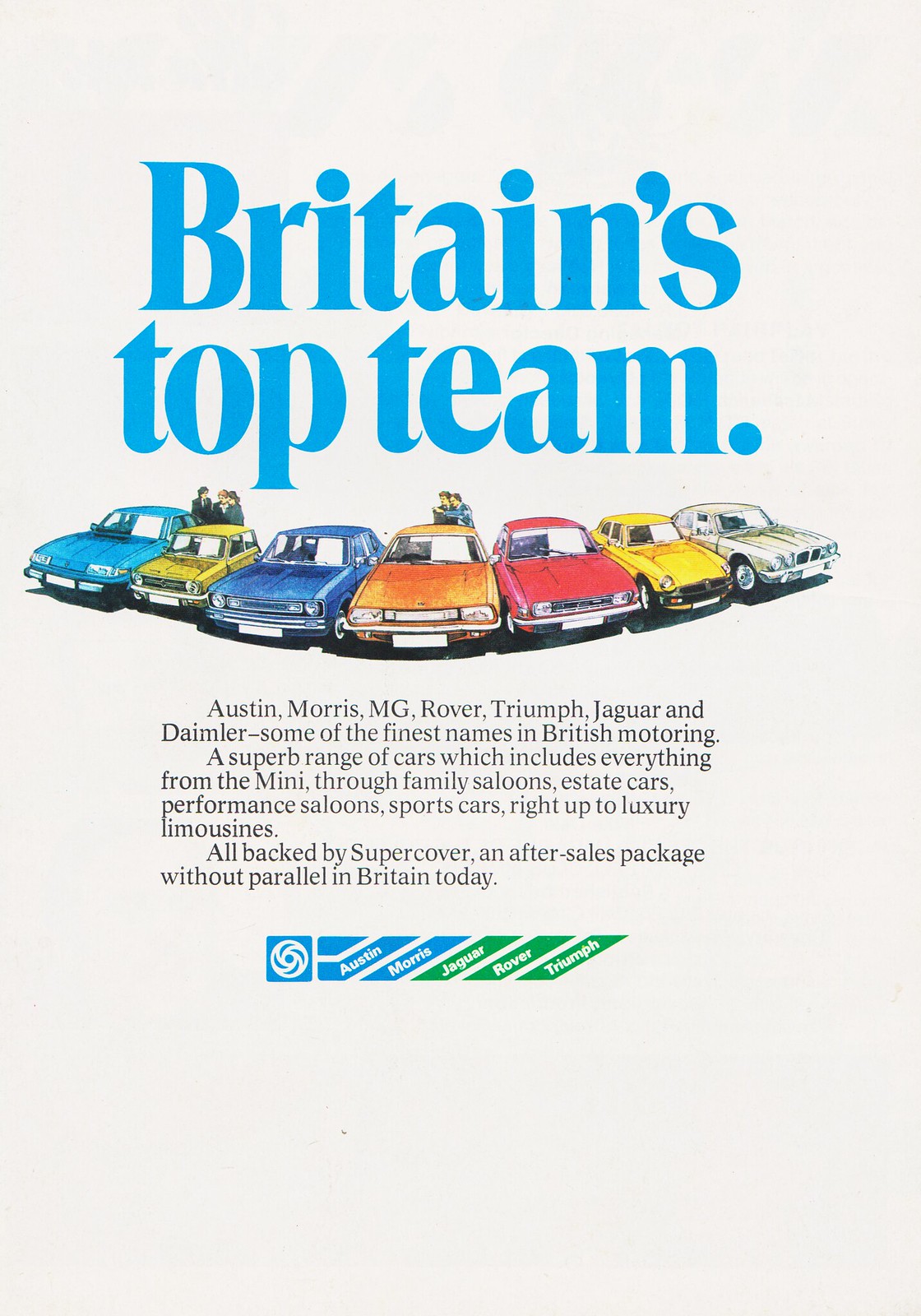The image features a vertically oriented advertisement with a white background prominently displaying the text in large blue letters, "Britain's Top Team." Beneath the headline, the front views of several old-fashioned cars are showcased in vibrant colors - blue, yellow, orange, red, and white. These cars are positioned in a slight arch formation, all facing forward. Surrounding the cars is a band of blue and green. Below the cars, there is text identifying some of Britain's finest motoring brands, including Austin, Morris, MG, Rover, Triumph, and Jaguar. The advertisement is styled like a computer-generated newspaper ad, celebrating the heritage and excellence of these iconic British car manufacturers.